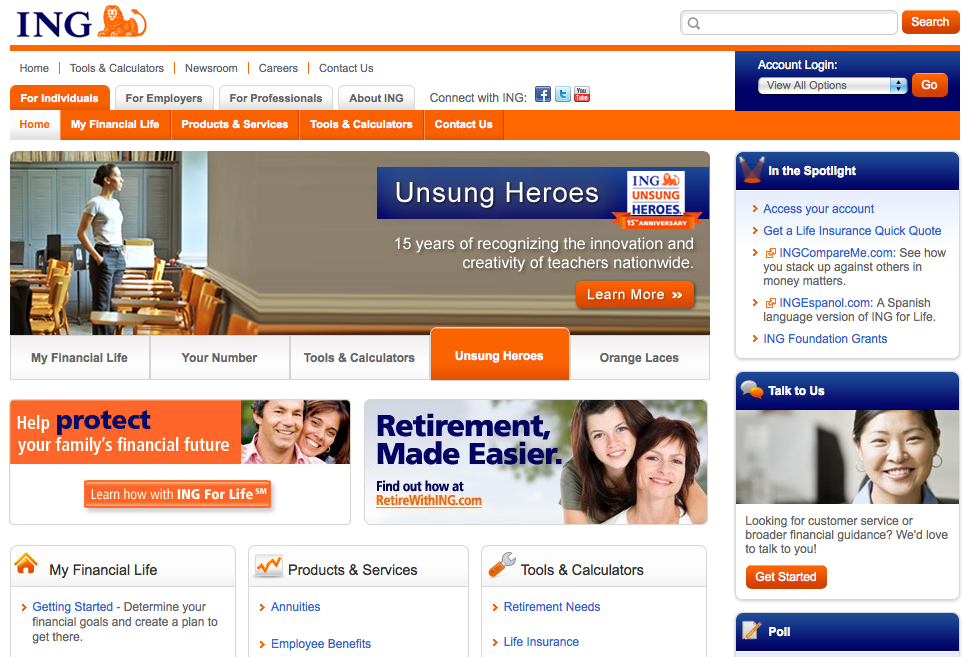The image depicts a website interface with a layout approximately 30% wider than it is tall. The background of the website is primarily white, with a distinct dark blue header at the top. In the top left corner of the header, bold capital letters spelling "ING" are displayed next to an orange lion logo. 

To the top right, there is a search bar featuring a gray magnifying glass on the left side of the input field. Adjacent to the search bar is an orange button with the word "Search" in white text at its center. 

Below this header, a horizontal orange bar runs across the width of the site. Underneath the bar, a series of menu items are laid out horizontally and aligned to the left, each separated by a vertical line. The menu items read: "Home," "Tools and Calculators," "Newsroom," "Careers," and "Contact Us."

On the right side of the menu, there is a section with a dark blue background labeled "Account Login." Below this heading is a selection box with "View all options" chosen by default. Adjacent to this box is an orange button displaying the word "Go" in white text.

Further down on the left side of the page, there is another set of tabs designated for different user categories: "For Individuals," "For Employers," "For Professionals," and "About ING."